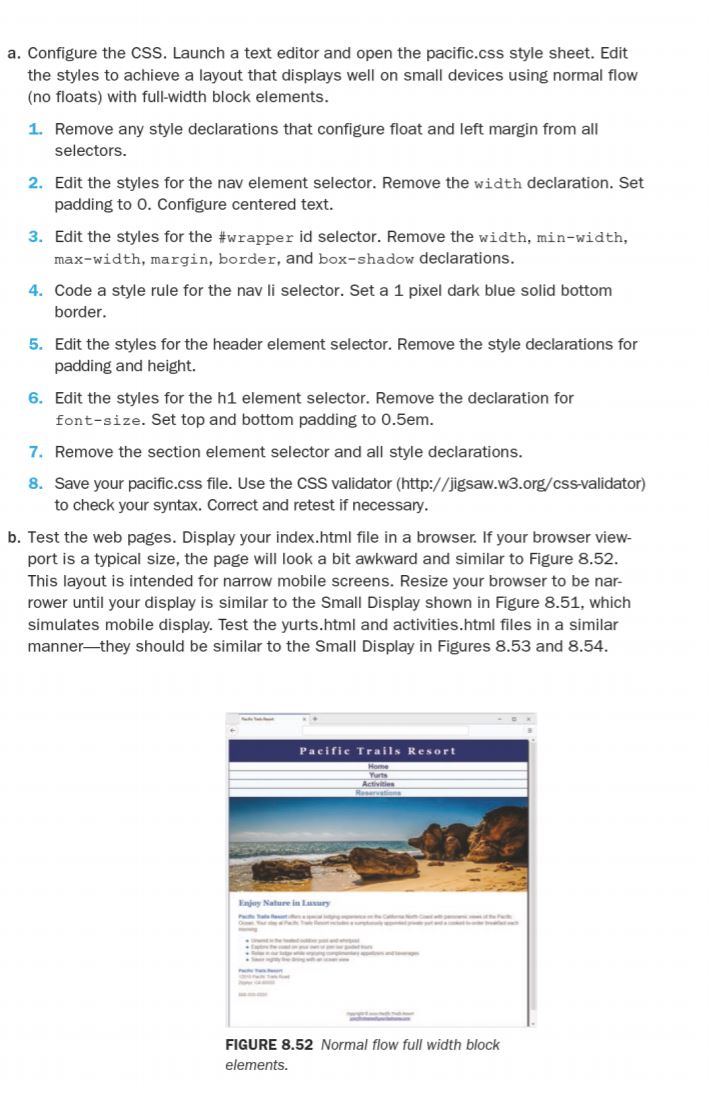This image displays detailed instructions for a technical activity related to website development. The content is text-heavy, featuring black text against a white background.

At the top, labeled "A," are instructions for configuring CSS. The steps instruct the user to launch a text editor and open the "pacific.css" stylesheet. It specifies editing the styles to create a layout suitable for small devices, focusing on normal flow with no floats and full-width block elements. Below this are eight numbered points, each providing specific instructions to ensure the website displays correctly on various screen sizes.

Labeled "B" further down, the instructions detail testing webpages. Users are to display the "inbox.html" file in a browser. If viewed on a typical-sized browser viewport, the page may appear awkward, similar to the illustration in Figure 8.52. This layout is optimized for narrow mobile screens. Users should resize their browsers until the display matches the small-screen simulation shown in Figure 8.51. Similar testing is required for the "yurts.html" and "activities.html" files to ensure they correspond to the small display examples in Figures 8.53 and 8.54, respectively.

Below these instructions, the image includes Figure 8.52, showcasing the "normal flow" layout with full-width block elements as it appears on a website.